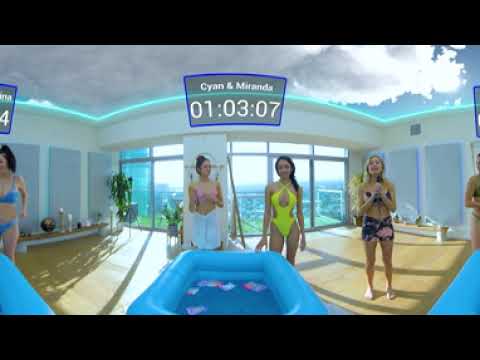In an expansive, roofless indoor space resembling a game room high up in a skyscraper, several women in swimsuits gather around a mildly filled blue inflatable wading pool. Centrally positioned in front of the pool are two women: one on the right, clad in a yellow one-piece bathing suit with cutout details, and another on the left, who sports a pink bikini top paired with a white skirt or towel. Nearby on the far left, a third woman stands partially visible, dressed in what appears to be a blue or purple bikini. To the right, a woman with blonde hair holds a microphone while dressed in a pink and blue bikini top with matching shorts. Cut off at the extreme right edge of the image is another woman, seemingly in a green bikini. Above these central figures, a floating blue-outlined transparent rectangle displays the names "Cyan" and "Miranda," alongside a timer reading "1 hour 3 minutes and 7 seconds." Flanking the scene are two additional blue wading pools, and in the background, large glass windows reveal a cityscape view. The photo is presented within a black-bordered rectangular frame, with an upper section showing clouds and a hint of blue sky with the Sun.